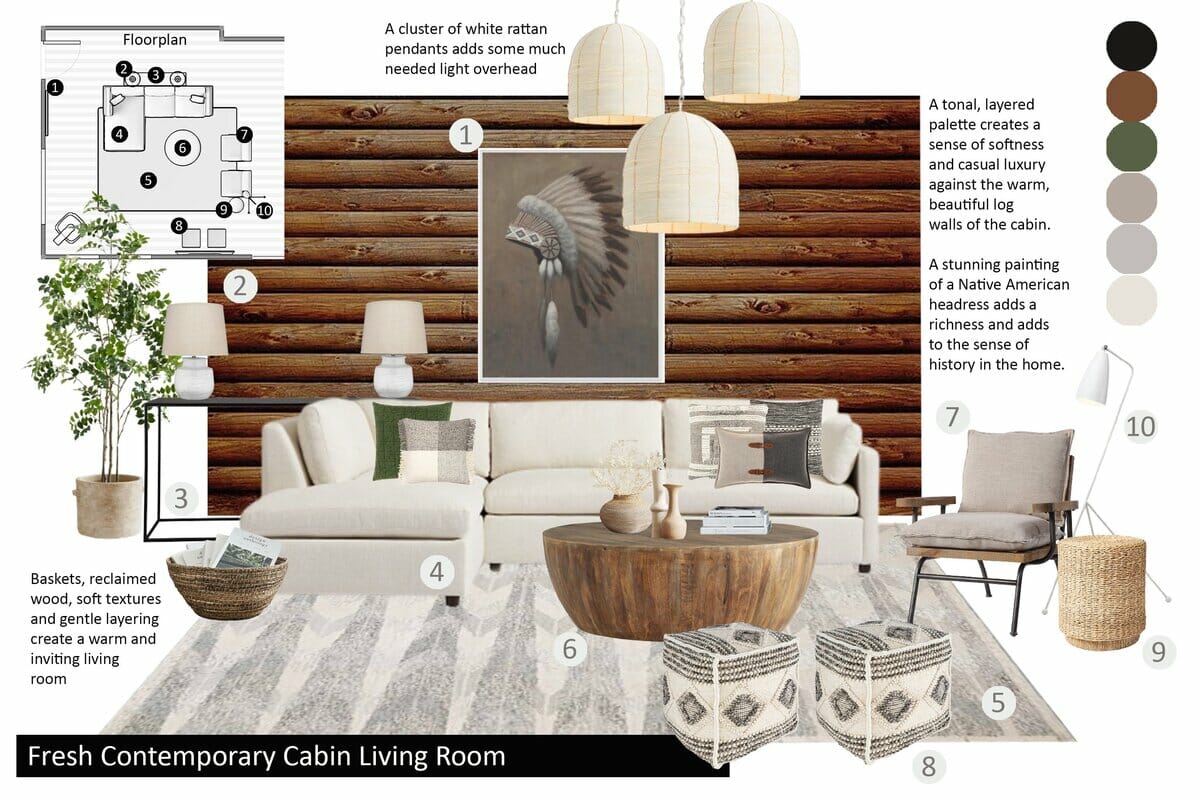This image is an advertisement demonstrating how to decorate a modern cabin living room. In the upper left corner, a gray box labeled "floor plan" shows an aerial sketch of the room, marked with brown-black dots and white numbers indicating item placements. The plan is slightly turned and some numbers don't align perfectly with the actual room layout.

To the right is a medium-brown log cabin plank wall adorned with a framed picture featuring a gray background and a Native American headdress, adding a sense of history and richness to the space. Centrally hanging from the ceiling are three light tan, rounded pendant lights, each corresponding to numbered items on the floor plan.

The main seating area includes a white L-shaped sofa with an accompanying chaise, and a simple rectangular table behind it, which hosts two lamps. Completing the cozy setup is a wooden coffee table resembling the bottom of a barrel, soft cube-shaped ottomans, and a potted plant for a touch of greenery.

At the top, a caption highlights how the cluster of white rattan pendants provides much-needed overhead light. On the right side of the image, six color swatches in black, brown, olive green, and three neutral tones display the palette used to achieve the space's tonal and layered look. The colors enhance the sense of softness and casual luxury against the warm log walls. 

Text at the bottom left reads "fresh contemporary cabin living room," emphasizing the modern yet inviting aesthetic. Additional captions mention how baskets, reclaimed woods, soft textures, and gentle layering contribute to the room's warm and inviting ambiance.